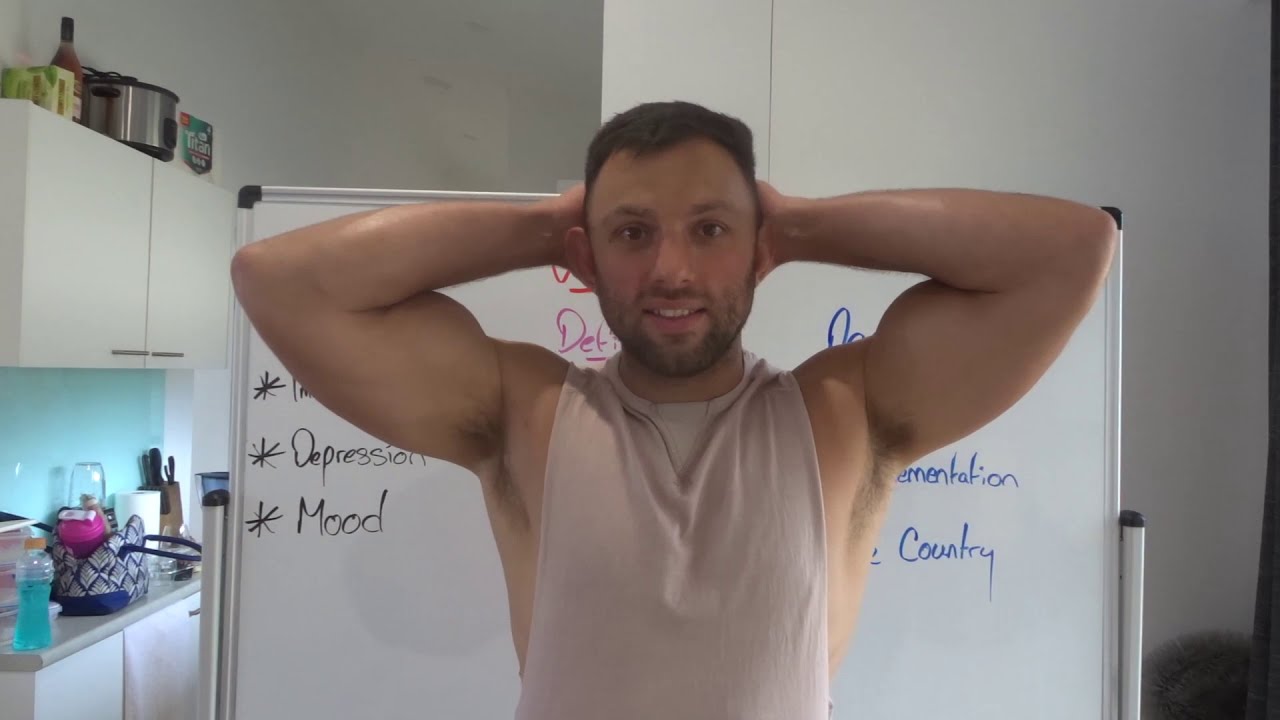The image depicts a well-built man with short brown hair standing in front of a mobile whiteboard in a brightly lit room, possibly a kitchen. He is facing the camera, smiling, and has his muscular arms raised with his hands behind his head. He is wearing a beige cut-off tank top. The whiteboard behind him, partly obscured by his body, features various handwritten notes, notably the words "depression" and "mood" in black, with asterisks next to them, red text in the center, and blue text on the right. To the left of the whiteboard, there are white cabinets with a bottle of red sauce and a silver crockpot on top. Below the cabinets is a mint green wall above a gray countertop, which holds a bright blue liquid in a bottle and what appears to be a lunchbox. The scene is well-lit with natural light, highlighting the man's figure and the details of the room.